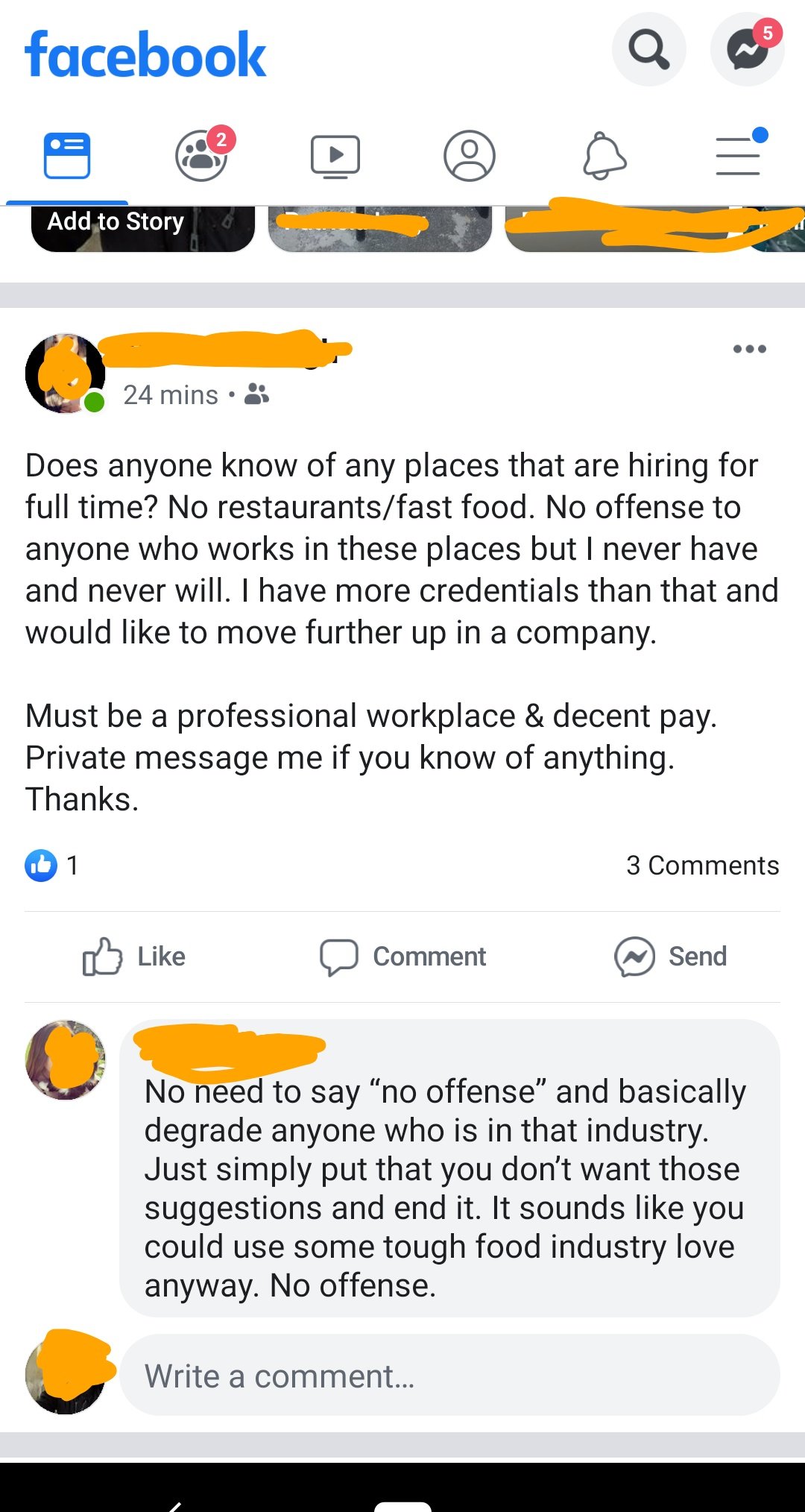The image shows a screenshot of a Facebook post viewed through the Facebook Messenger interface. In the top left corner, the word "Facebook" is prominently displayed in blue. Adjacent to this, there are two light gray icons: a magnifying glass symbolizing search functionality, and a text bubble overlayed with a number "5," indicating five unread instant messages. Beneath these icons, a light gray border spans the screen.

The screenshot has been edited with an orange marker filter to blur out profile pictures and names, rendering them unreadable. Despite this, the text of the Facebook post remains visible. It reads:

"24 minutes ago:
Does anyone know of any places that are hiring for full-time? No restaurants/fast food, no offense to anyone who works in these places, but I never have and never will. I have more credentials than that and would like to move up further in the company. Must be a professional workplace and decent pay. Private message me if you know anything. Thanks."

Below the post, it notes the existence of "three comments" and displays engagement options including "Like," "Comment," and "Send," all in gray text. A visible comment from another user criticizes the original post:

"No need to say 'no offense' and basically degrade anyone who is in that industry. Just simply put that you don't want those suggestions to end it. It sounds like you could use some tough food industry love anyway, no offense."